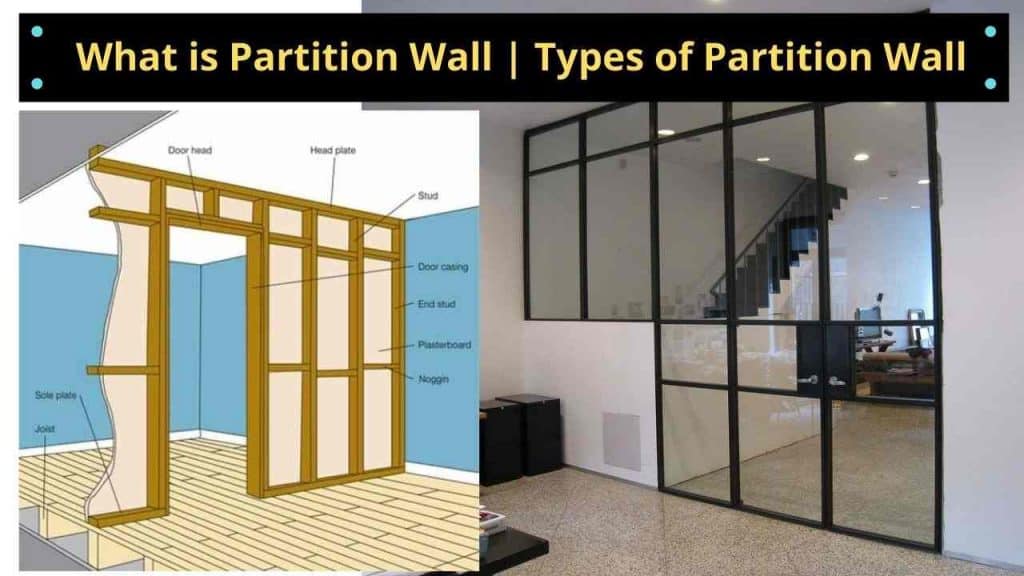The composite image titled "What is a Partition Wall? Types of Partition Wall," showcases a detailed comparison between the structural diagram of a partition wall and an actual finished photo. The upper border of the image contains a black background with the title written in yellow text, flanked by four blue dots. 

On the left, the diagram illustrates the different components of a partition wall, albeit with some labels being too small to read clearly. Visible labels include "door head," "head plate," "stud," "door casing," "end stud," "planter board," "nogging," and "side plate." The partition wall structure in the diagram features a brown frame standing on a tannish yellow base with a white ceiling.

To the right is a photograph of the completed partition wall, which features clear glass panels within the brown framework. This wall separates an interior space, revealing parts of the room behind it. Through the glass, you can observe a pair of black stairs leading upwards, two doors on the right, and other room details, suggesting an office or residential setting. The floor appears to be made of granite or marble, with white surrounding walls and some black objects providing contrast. This side-by-side presentation effectively illustrates both the construction phase and the finished state of a glass partition wall.